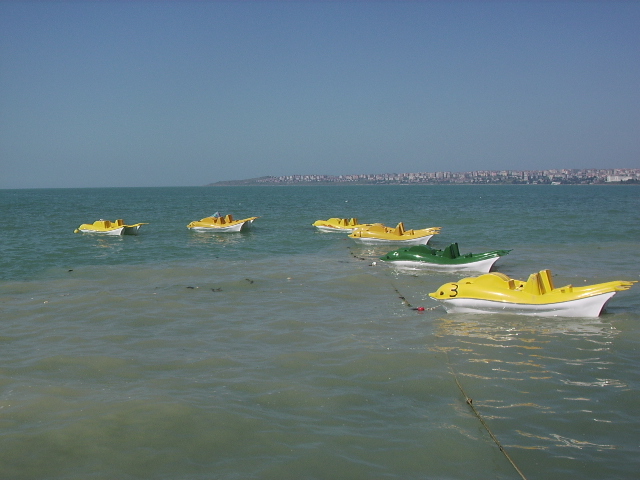The image depicts a serene coastal scene, wider than tall, capturing a shallow bay with clear, calm water that transitions from a murky brown near the shore to a bluish-green further out. Occupying about two-thirds of the water area, the surface appears shallow enough to reveal the sandy bottom near the paddle boats, which are tethered together by a rope leading from the right side of the image. There are six paddle boats in total: five are yellow and one is green. The yellow boats each feature two seats and whimsical faces painted on their fronts, complete with eyes and ears, creating a playful appearance. These boats are arranged close to the shore, with two extending slightly further into deeper waters. On the right-hand side, a brown peninsula stretches into the bay, speckled with white dots that likely represent buildings. Farther in the background, beyond the silky blue-green haze of the water, a row of gray buildings can be discerned, adding urban context to the otherwise natural setting. The sky overhead is a clear, medium blue, free of clouds and bathed in sunlight, encapsulating the overall tranquility of the scene.